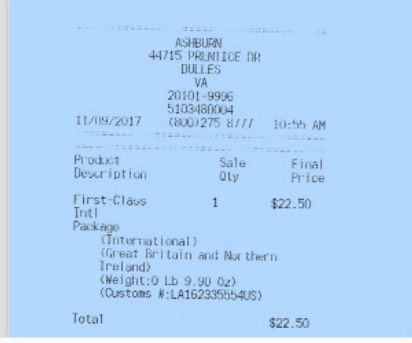This photograph captures a blue-colored square receipt. The heading of the receipt reads "Ash Byrne" followed by the address "44715 Prentiss Drive, Dulles, Virginia, 20101-9996." Beneath the address is a number, "5103-480004." The receipt is dated "11-09-2017" with a timestamp of "10:55 AM." Detailed sections include columns for the product description, sales quantity, and final price. The item purchased is listed as a "First-Class International Package." The buyer bought one package for a total cost of $22.50. Additionally, the receipt specifies that the destination for the package is Great Britain and Northern Ireland, affirming the total transaction amount of $22.50.